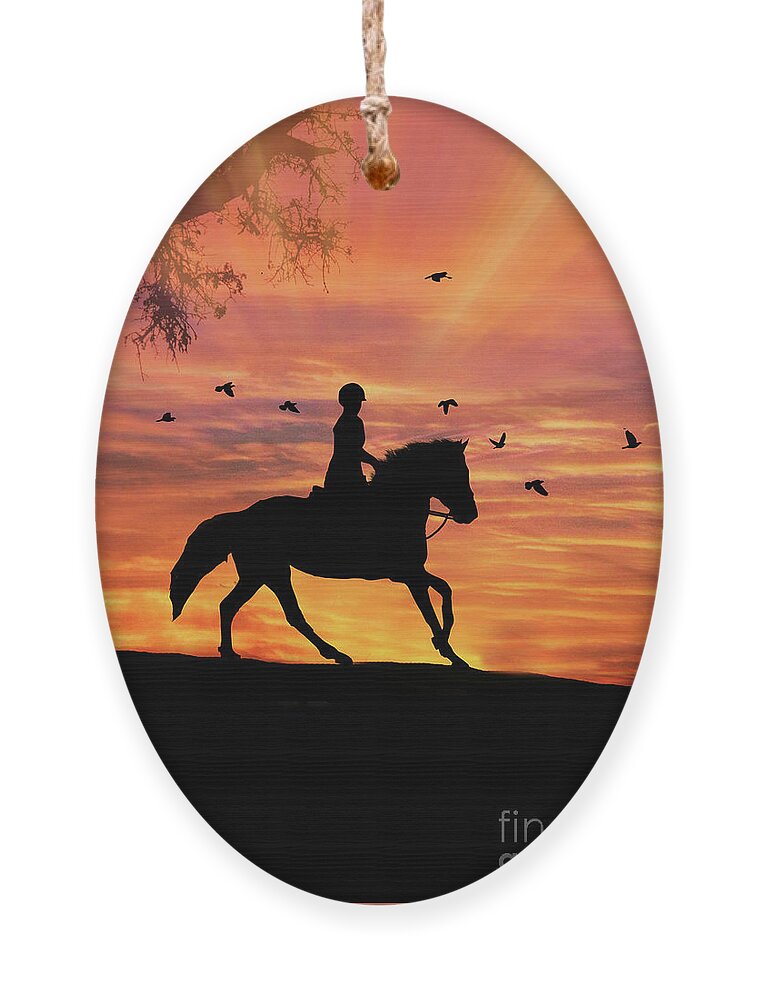The image depicts an oval-shaped wooden medallion or decoration, likely designed for hanging in a rustic or country setting like a barn or a country house. It hangs from a rope threaded through a hole at the top, secured by a knot. The central artwork within the medallion is a striking silhouette of a person riding a galloping horse, both appearing in black against a vivid background featuring the warm hues of a setting sun in orange, yellow, and touches of purple. Additional details include birds flying in the sky behind the rider and some tree limbs extending into the frame from the upper left. The ground beneath the horse is rendered in solid black, and there are faintly visible letters "F-I-N" at the bottom right, partially obscured. The overall scene evokes a sense of motion and majesty, capturing a timeless equestrian moment.